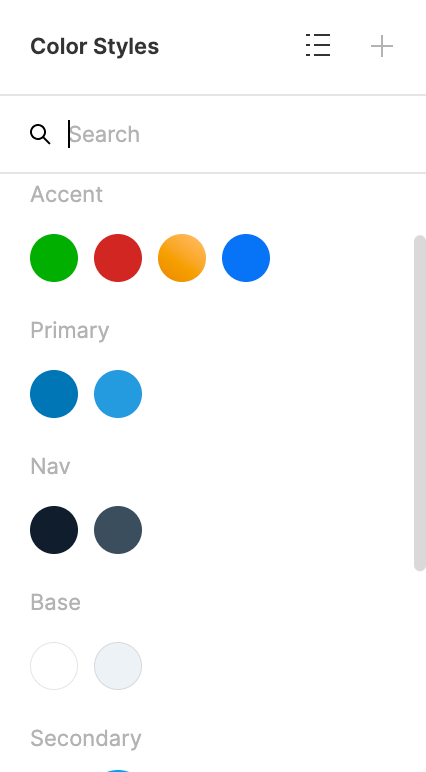The image appears to be a screenshot from a phone, displaying a user interface related to color customization. The visible section excludes the outer borders and the very top portion of the phone. 

At the top, the text "Color Styles" is prominently bolded in black. To the right, there are three horizontal lines each accompanied by three short vertical lines, with slight spacing between them, suggesting a menu or settings icon. Following this is a faded gray plus sign.

Beneath this header is a thin gray dividing line, under which there is a search bar. The search bar is a white rectangular field with a magnifying glass icon preceding the word "Search".

Below the search bar is the section labeled "Accent." In this section, there are four color circles: green, red, orange, and blue. The next section is labeled "Primary" in light gray text, featuring two circles, one dark blue and the other light blue.

Following "Primary" is the "NAV" section, showcasing two color circles: one black and the other appearing to be an aqua blue.

The "Base" section is listed next, displaying a white circle and a light gray circle. At the bottom of the image, partially visible, is the "Secondary" section, which shows the tip of a blue circle.